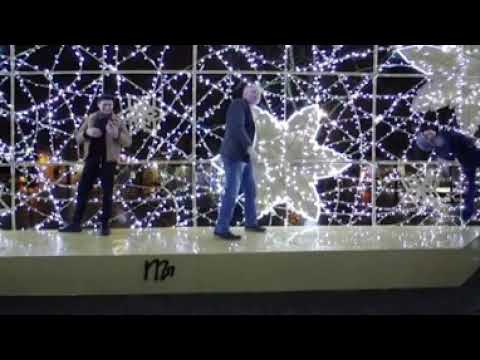The image captures a festive winter scene, likely during a Christmas or holiday event. Two men stand on a reflective, stone-like or marble platform adorned with numerous Christmas lights and white star-shaped light decorations. The man on the right is middle-aged, wearing blue jeans, dark shoes, and a blue long-sleeve sweater. He is bald and gazes to the right. The man on the left wears a cream-colored jacket over a black shirt and black pants, and he is seen checking his cell phone with his left hand. The setting is dark with the bright, blue-white string lights illuminating the scene. The background suggests a residential neighborhood, possibly hinting that the event is community-driven. The overall atmosphere appears to be a cheerful winter night with a significant emphasis on holiday decorations and lights.